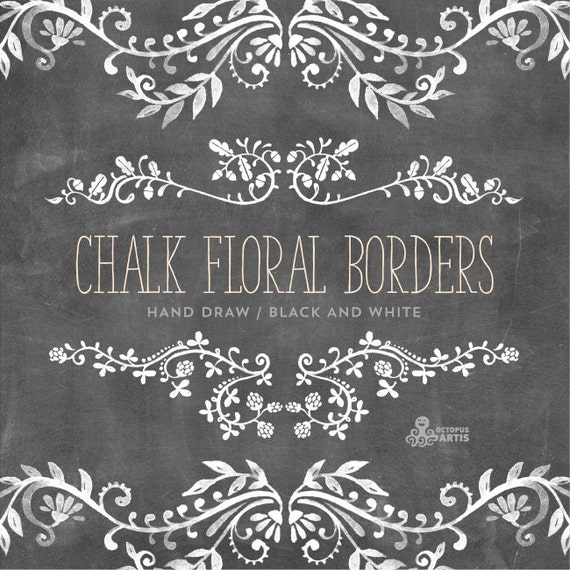The image resembles a cover for a book, poster, or ad, featuring a primarily black and white design with a dark, chalkboard-like background exhibiting shades of gray and chalk residue. Prominently displayed in the center is the title "Chalk Floral Borders," written in light yellow capital letters, mimicking chalk writing. Just below the title, the subtitle reads "Hand Draw / Black and White" in smaller, fainter letters. The design is framed by intricate floral borders: larger, elaborate vines with leaves and flower buds at the top and bottom edges, mirroring each other, and smaller versions of these intricate patterns placed towards the interior. These plant motifs start from the edges and symmetrically wind towards the center. At the bottom right corner, the logo showcases a small gray octopus with the text "Octopus Artist" beside it, further enhancing the old-school, silent movie text screen aesthetic.